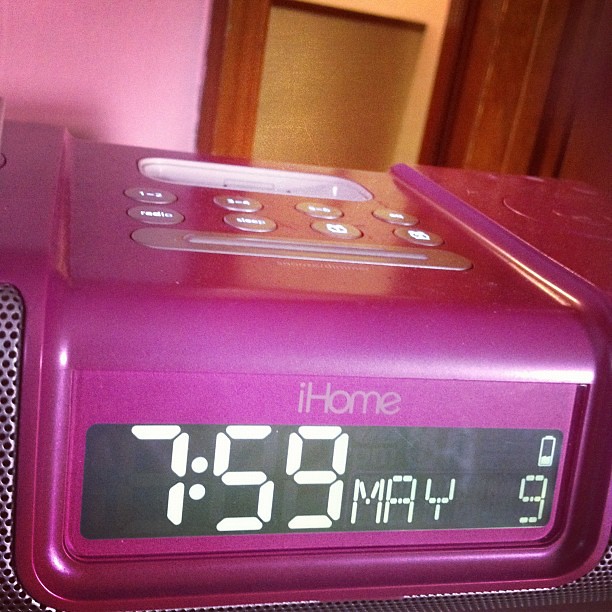The photograph showcases a digital clock radio made by iHome, predominantly colored in a purplish-pink hue. The device rests against the backdrop of a pink room adorned with white wooden molding and a wooden door. The iHome features a prominent LCD screen on the front, displaying the time "7:59," the date "May 9th," and a battery icon indicating about one-third power remaining. The top of the device is populated with various buttons that have white inscriptions, including functions such as "Radio" and "Sleep." A handle, currently flat but designed to be lifted, sits prominently on the top for convenient portability. The speaker sections, characterized by silver U-shaped parts with holes in them, flank the display screen which reads "iHome" in gray font above the digital readout. The overall impression is of a functional yet stylish digital clock radio set within a homely environment.